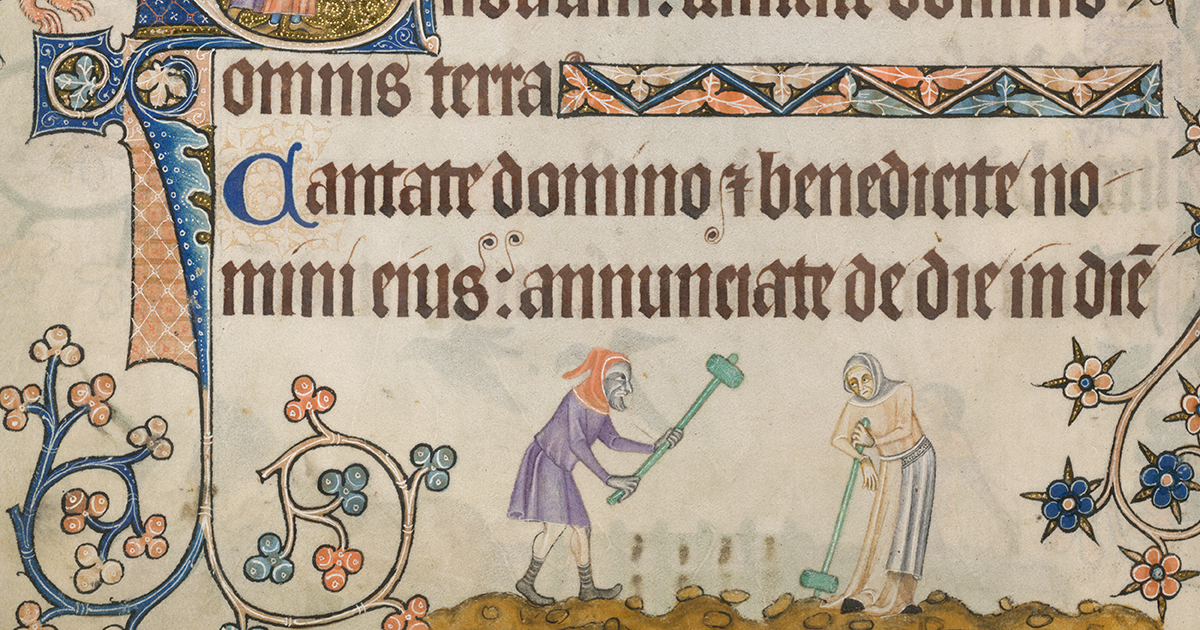This image appears to be an intricate, hand-drawn and colored depiction resembling a medieval illuminated manuscript. The artwork features detailed designs throughout, including a prominent large letter that integrates into the border and transforms into what looks like a tree root. Along the border, various abstract patterns and colorful figures can be found. Notably, there's a blue-stemmed flower with vibrant orange and blue petals, adding a splash of color to the composition. At the bottom of the page, two peasants, depicted with hammers in hand, are laboring over the brown soil, which is visibly breaking away under their strikes. The centerpiece of the image is a beautifully rendered gothic script in Latin, reading "Canta Domino Benecito." The overall style and meticulous detail suggest this piece is not merely a design but a richly illuminated page, reminiscent of historical manuscripts.